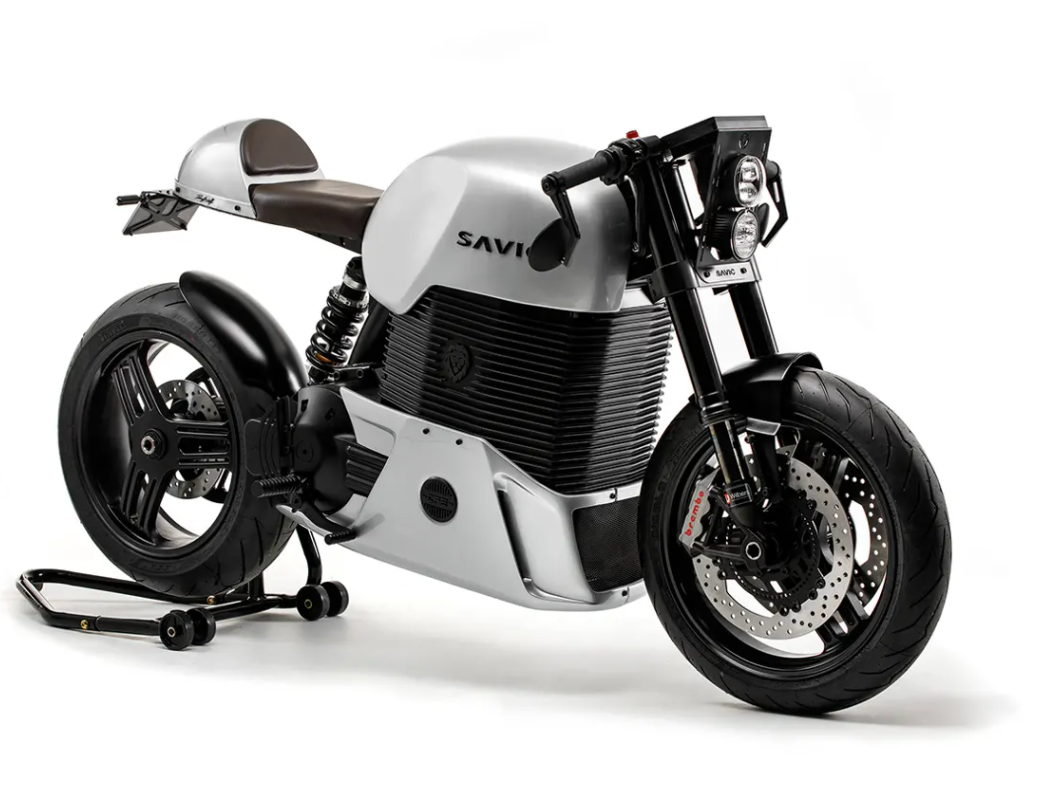The image features a highly detailed, futuristic motorcycle set against a pristine white background, which ensures all attention is drawn to the bike itself. The motorcycle embodies a blend of retro and modern design elements, resembling something straight out of Tomorrowland. The bike's body is primarily black and silver, with bulky and robotic contours that contribute to its aerodynamic and ergonomic appearance. 

Distinct features include two prominent front headlights, a pair of fat, heavy tread tires, and a unique black and brown leather seat. The seat itself is raised, with no visible frame connecting the back tire and the seat except for a shock absorber. Text near the top of the bike reads "SAVI," though it is partially obscured by the handlebars. Additionally, there is red text around the wheel area spelling "Bramby" and a license plate on the front right side of the motorcycle. 

The motorcycle is slightly suspended with the rear wheel elevated by a small jack or possibly a set of training wheels which are part of a black contraption. Across various parts of the bike, silver gears and trimmings are visible, amplifying its intricate mechanical design. Despite its detailed construction, the motorcycle has an appearance that suggests it is more of a conceptual model than a functional vehicle.